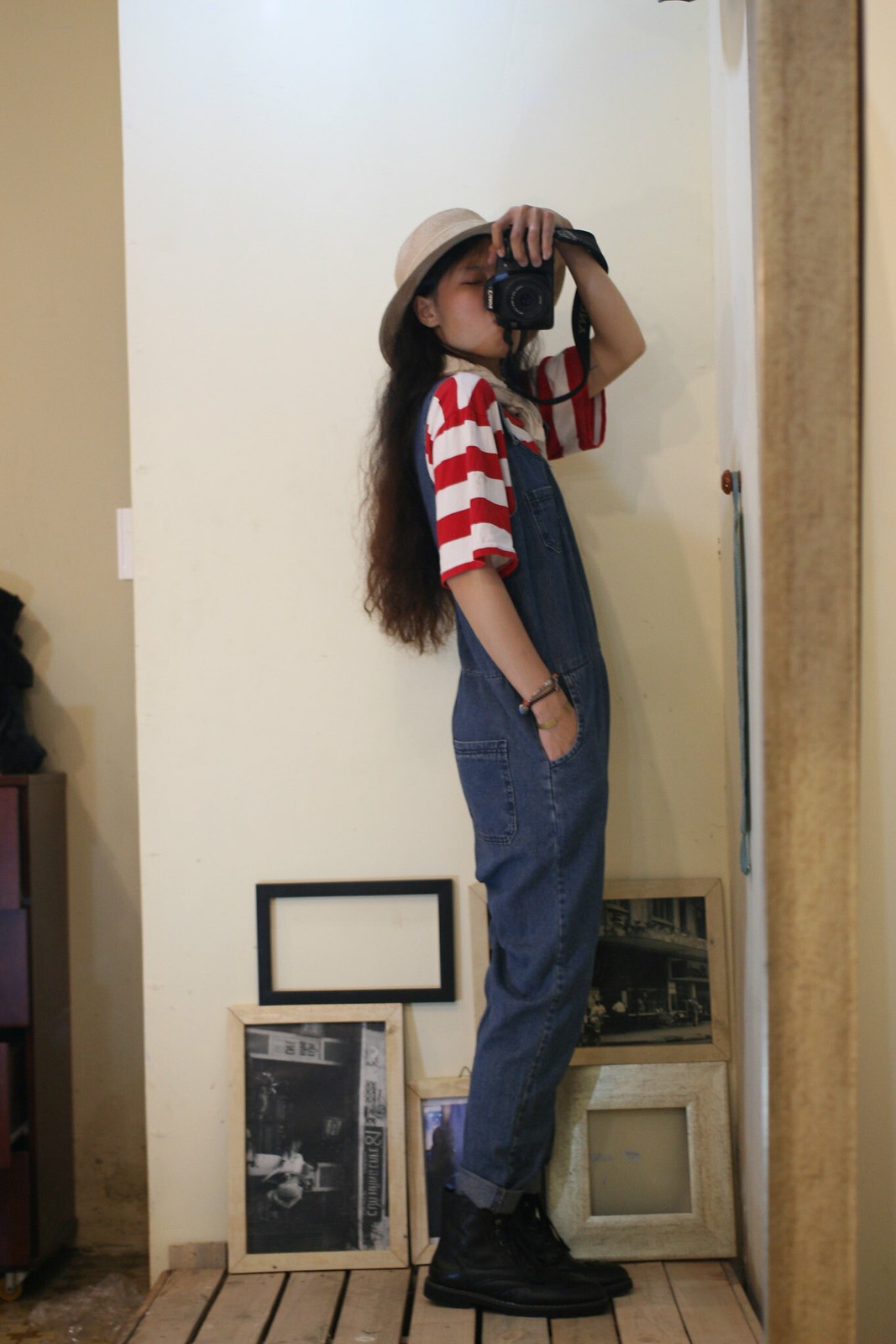This is a detailed photograph featuring a young, slender girl with long brown hair, possibly of Asian descent, standing on natural wood slats in front of a white wall. She is partially in profile, facing the right, wearing a light-colored hat, denim overalls rolled up at the ankles, a red and white striped short-sleeved shirt, and black boots. Her left hand, adorned with a bracelet, holds a black vintage camera with a strap, positioned in front of her face, and her visible eye is closed as if she is about to take a photo. Her right hand is casually tucked into her pocket. Behind her, there are several photographs—some framed, some not—leaning against the wall. These include a mix of vintage images at the bottom and empty black and white frames. The setting is minimalistic, with a brown door visible to the side and no carpeting on the wooden floor, enhancing the vintage, artsy atmosphere.